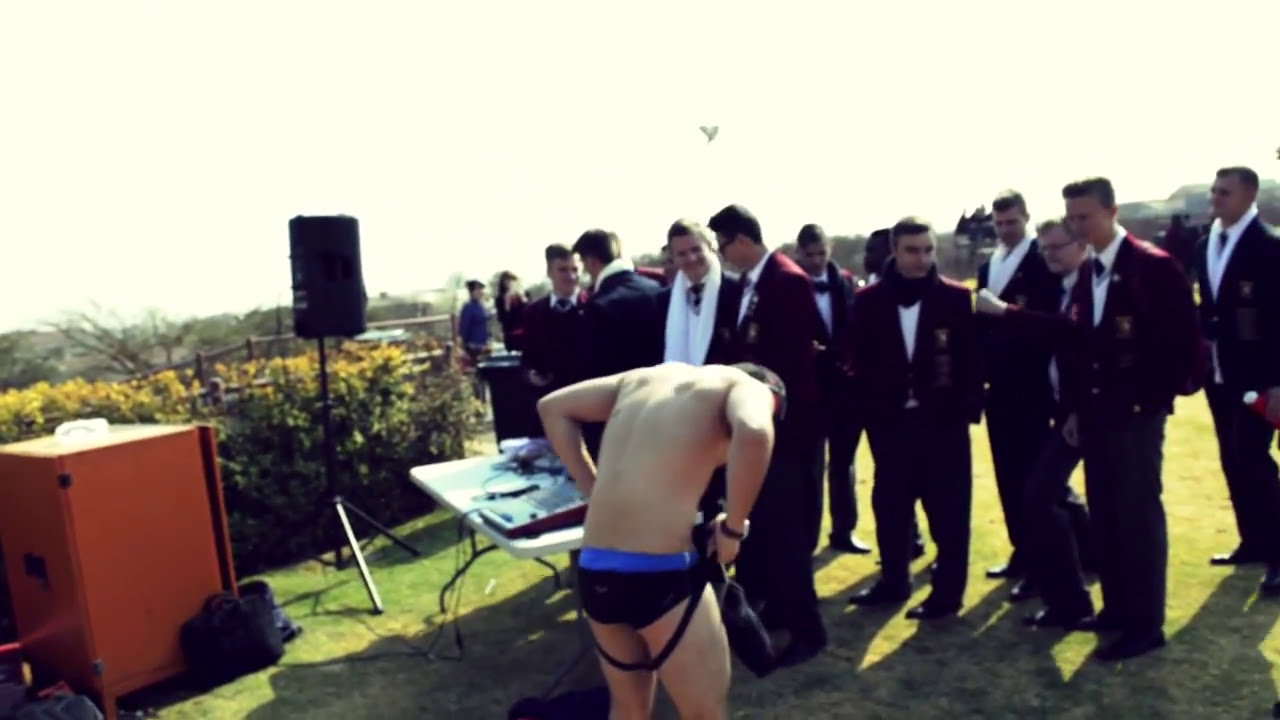In a shady backyard setting, a peculiar scene unfolds with a group of young men, likely college graduates or fraternity members, all dressed in coordinated attire. They don dark red blazers, white dress shirts, black bow ties, and dark gray pants paired with matching shoes, exuding an air of formal sophistication. All individuals in the image are white-skinned, smiling subtly, their attention divided but none fixated on the central figure except one.

The focal point is an almost-naked man, clad only in underwear with a blue waistband and two straps hanging down his thighs. He appears to be adjusting or pulling up a pair of additional black trunks. In front of this peculiar figure is a white table with some unidentified items on it, alongside a speaker mounted on a stand to the left. Further left stands a brownish-orange cabinet with a small white object on top. The backdrop is dotted with large dandelion-like flowers on tall green stems, adding to the quirky ambiance of the scene.